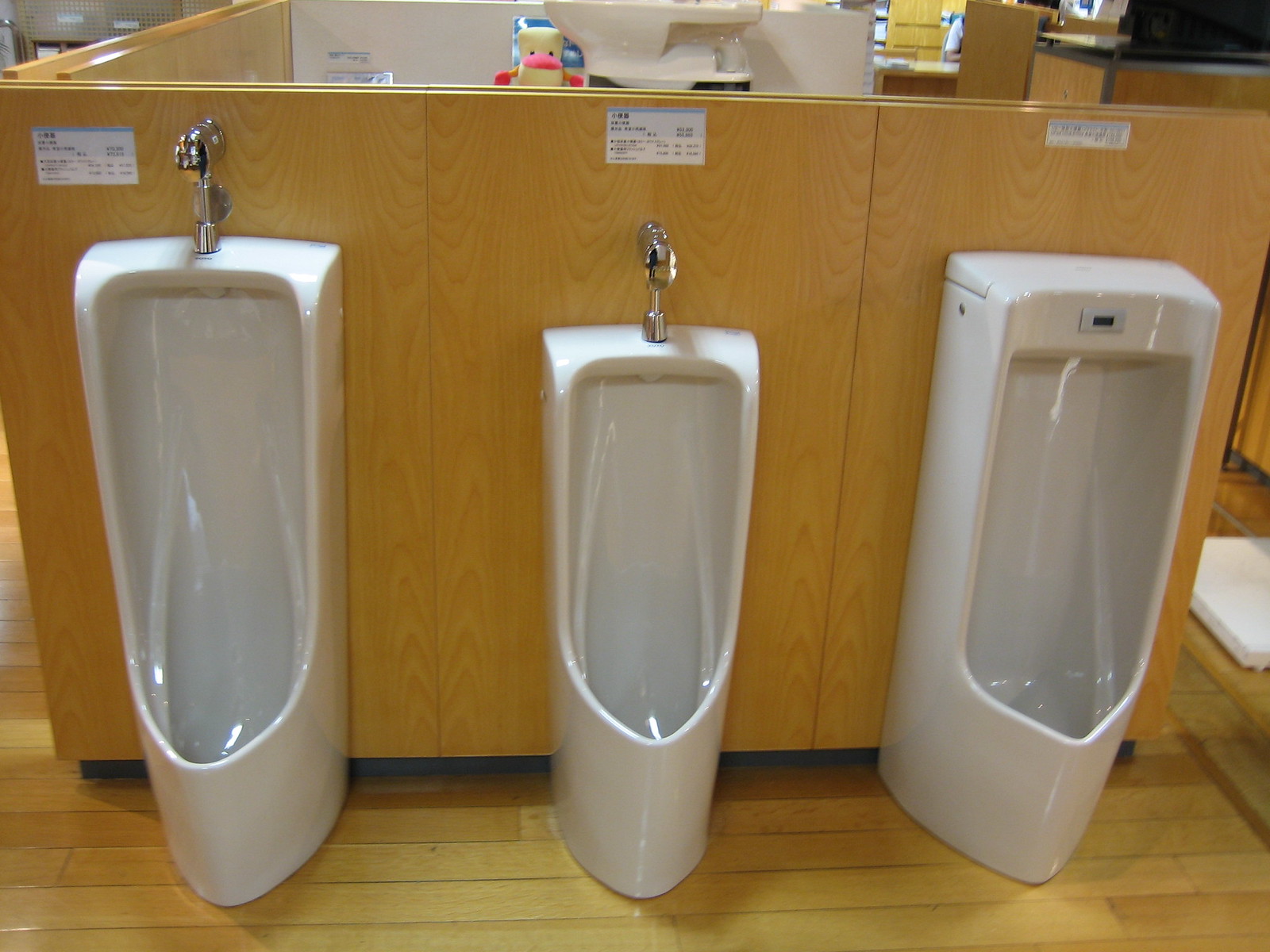In this image, we see a showroom display in a hardware store featuring three white porcelain urinals, each mounted against individual wooden boards. The setup gives an open, non-traditional bathroom feel. The urinals are aligned in a row, with the left and right urinals being of the same height, while the middle one is noticeably shorter. The left and middle urinals have visible plumbing fixtures extending from the top, whereas the right urinal features a sleek, black sensor box. Sitting atop the wooden dividing wall of the middle urinal is a toy duck, whimsically peering over. Above each urinal, white pieces of paper display information, likely including prices, as these units are for sale. The floor below is wooden, and in the background, various kitchen items are visible, emphasizing the store's diverse inventory.